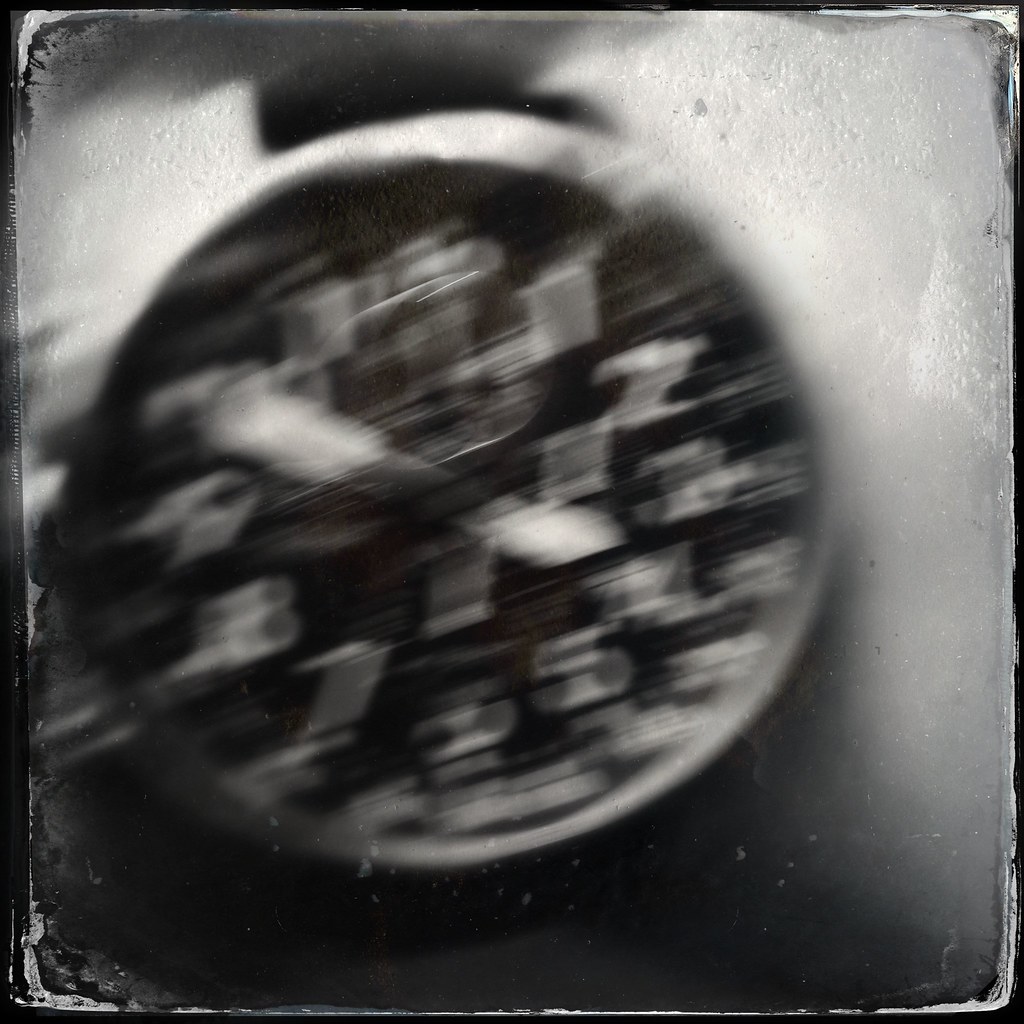In this highly blurred vintage photograph, the central focus appears to be a round object, potentially the face of a wall clock or a watch. The image is so obscure that details are challenging to discern, but there are noticeable white block numbers encircling the round face, not in Roman numerals. Two faint white hands seem to be present, pointing to various positions on the clock or watch. Above this round face, there is a subtle hint of a dark strap or perhaps a shadow, adding some depth to the image. The darkest region in the photo lies beneath the round object, fading into a near-black shadow. The background suggests that it might be positioned against a table, though this is not clear due to the overall blurriness of the photo.